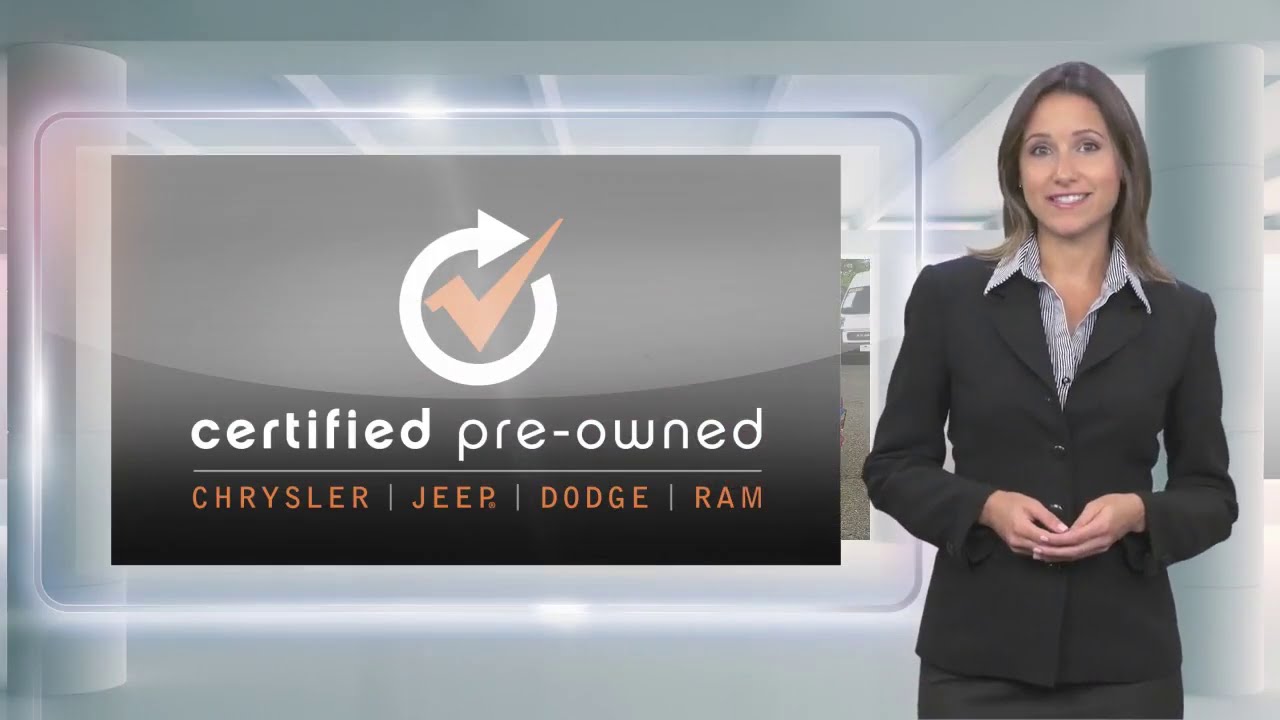The image depicts a still from what appears to be a commercial for a car dealership, focusing on Certified Pre-Owned vehicles from Chrysler, Jeep, Dodge, and Ram. On the left-hand side of the image, there is a distinctive black rectangular card with a silver lining and curved corners, featuring a gradient that transitions from dark gray at the bottom to lighter gray at the top. Prominently displayed on the card are the words "Certified Pre-Owned" in white, followed by "Chrysler, Jeep, Dodge, and Ram" in orange. At the top of the card, there is a white circle with a circular arrow and an orange checkmark inside, drawing attention to the certification.

In the rightmost part of the image, a woman is standing in front of one of two large white pillars, beneath a white awning. She is dressed in a professional black suit jacket over a collared, black-and-white striped shirt. Her long brown hair falls gracefully to her shoulders, and she has a warm smile, showcasing her white teeth. Her demeanor is confident and professional, suggesting she is effectively presenting the certified vehicles. The background of the image features a greenish hue, and to her left, behind the card, one can spot faint images of the cars being advertised. The scene radiates a polished, CGI-enhanced look typical of high-quality dealership advertisements.